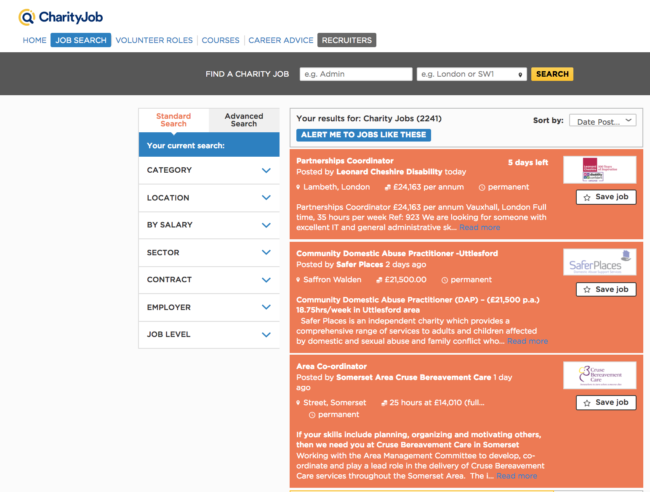This screenshot from the Charity Jobs website displays a user interface focused on facilitating job search within the charity sector. 

At the top right corner, there's a prominent magnifying glass icon encircled in yellow, signifying the search function. Beside it, the website's name "Charity Job" is displayed in navy blue font, ensuring brand visibility. 

Just below, a navigation bar is present with several options in blue font: "Home," "Job Search" (highlighted in a blue rectangle with white text), "Volunteer Roles," "Courses," "Career Advice," and "Recruiters" (highlighted in a dark gray rectangle with white text). 

A large central rectangle encourages users to "Find a Charity Job," featuring a search bar with placeholder text "e.g., admin" and a location field with "e.g., London." The search button is conspicuously designed in bright yellow.

Below this, job listings are visible, emphasized with an orange highlight and white font displaying options like "Star," "Save Jobs," and "Save Places." To refine the search, several filters are available on the right side of the page, including "Category," "Location," "Salary," "Employer," and "Job Level," each featuring drop-down arrows in varying shades of blue for easy navigation. The well-organized layout is designed to streamline the process of finding a job in the charity sector.